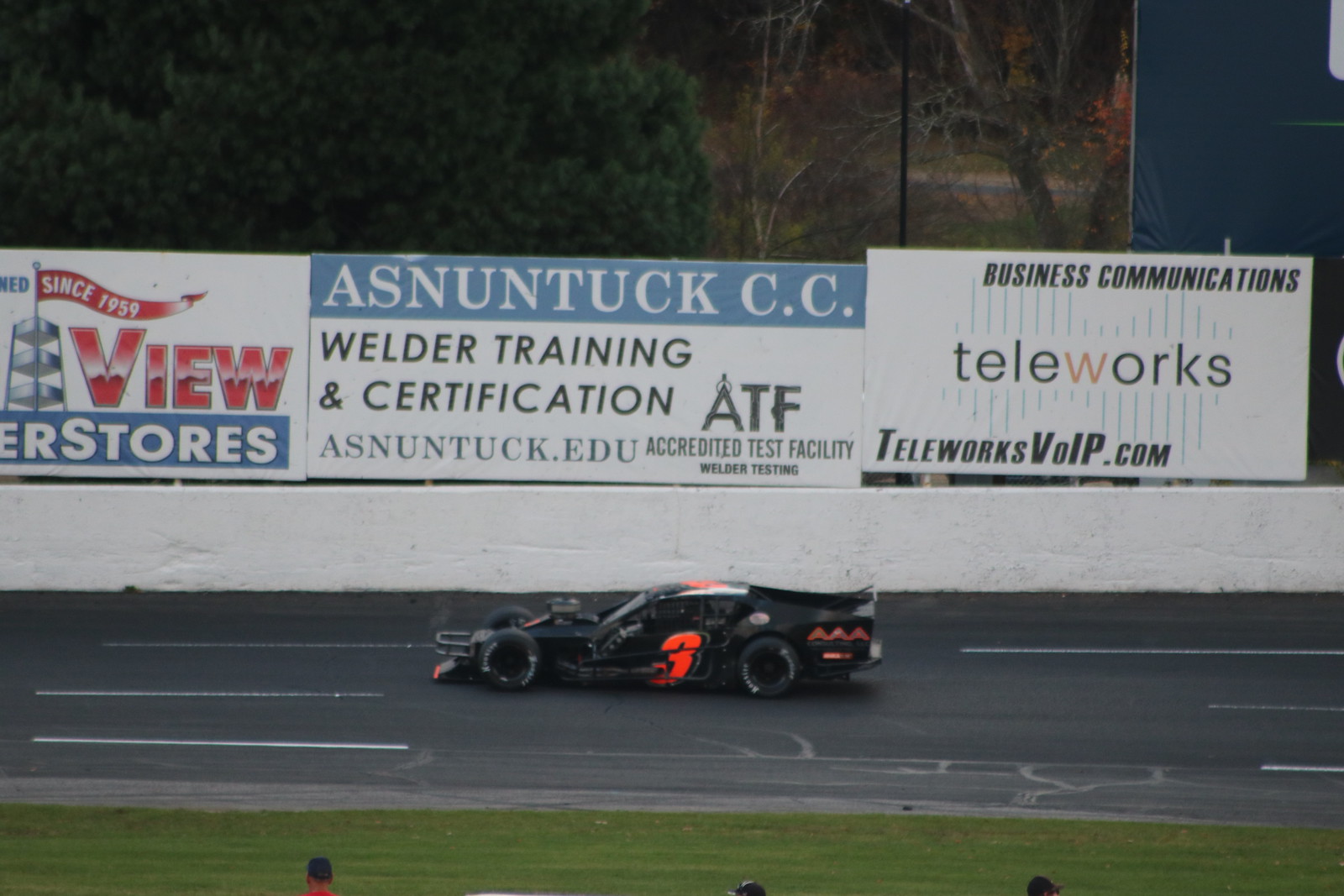The photograph captures a dynamic moment on a racetrack, focusing on a sleek black race car with a prominent, bright red number three on its side. The photo, taken from a slightly elevated angle, frames the car in full action as it speeds down the race strip. Surrounding the track, noticeable details include the bright green grass indicating a summertime event, and the heads of spectators peeking above the railings.

In the background, three distinct advertising signs can be seen along the track's sidewall. The leftmost sign, partially visible, features the words "since 1959" and "VIEW" in red, followed by "stores" though it's partially cut off. The middle sign advertises "ASNETUC CC Welder Training and Certification," alongside the accredited website info for ASNETUC. The rightmost sign promotes "Business Communications TeleWorks," with a mention of TeleWorksVOIP's website for voice-over internet protocol services. Beyond the signs, dark buildings loom, casting ambiguity on the time of day.

Overall, the scene vividly captures the intensity and speed of the race, highlighted by the stark details of the car, the colorful advertisements, and the energetic environment of the racetrack.